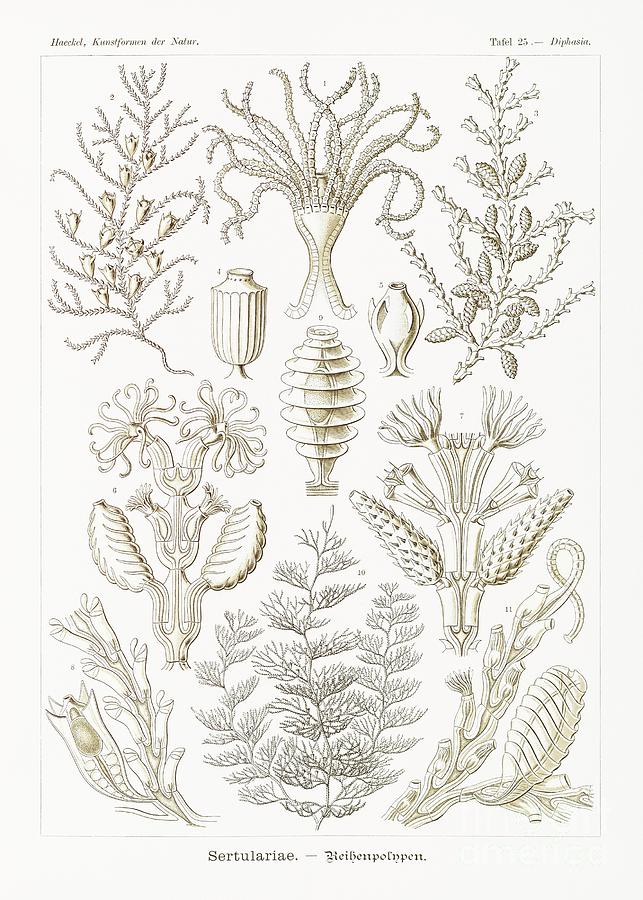The image appears to be a detailed botanical diagram set against a light pink background, showcasing an array of intricate plant-like drawings in dark brown and black hues. Central to the illustration is a plant with long, rope-like tendrils emerging from a vase-like structure. Surrounding this focal point are various plants, including trees, bushes, unique branches, and some elements that resemble underwater coral or bird-like forms. The upper left corner features tendrils with buds, while the upper right displays a stem with pine cone-like structures. At the bottom of the diagram, a fern-like plant is depicted. Scattered throughout the image are scientific names, though they are often difficult to read.